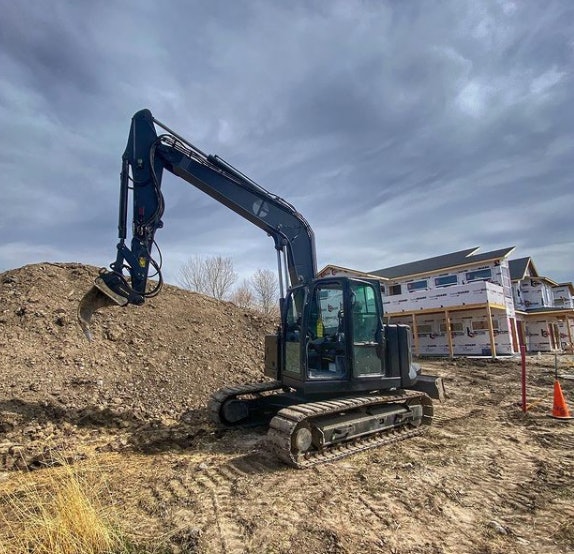The image captures an outdoor construction site under a stormy, overcast sky filled with expansive gray, puffy clouds. In the foreground, a blue bulldozer with an extended arm and claw is engaged in excavating a large dirt pile. The bulldozer, featuring treads at the bottom and a cockpit, appears alongside a dirt mound, indicative of ongoing site preparation. Adjacent to the machinery lies a yellow or orange traffic cone. The background showcases a series of newly constructed two-story houses or townhomes. These buildings are at an intermediate stage, exhibiting wooden structures with black roofs and wrapped in white insulation, awaiting further construction. The lower angle of the mobile photo provides a vivid view of the bustling activity at this developing site.